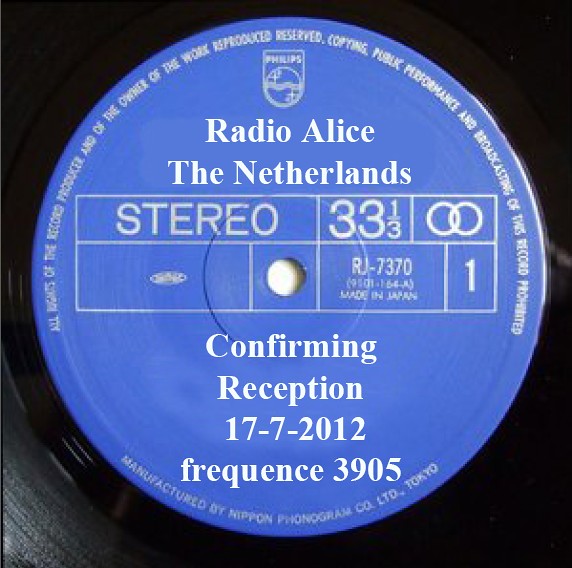This color photograph is a close-up of a record, showcasing the circular blue label at its center against the shiny black vinyl backdrop. The label, a sky blue circle with a small hole in the center, is adorned with white text. Encircling the top edge of the sticker is fine print, and at the top-center, there's a Philips logo featuring an earth badge and the company's name. Below this logo, the label reads "Radio Alice, The Netherlands," followed by a large rectangular section divided into smaller rectangles. These rectangles contain various inscriptions such as "Stereo," "33 1/3," interjoined circles denoting stereo sound, and numerical codes, including "RJ 730 70." Towards the bottom of the label, it states "Confirming Reception, 17-7-2012, Frequency 3905." The image reveals only part of the surrounding black vinyl, emphasizing the intricate details on the blue label.